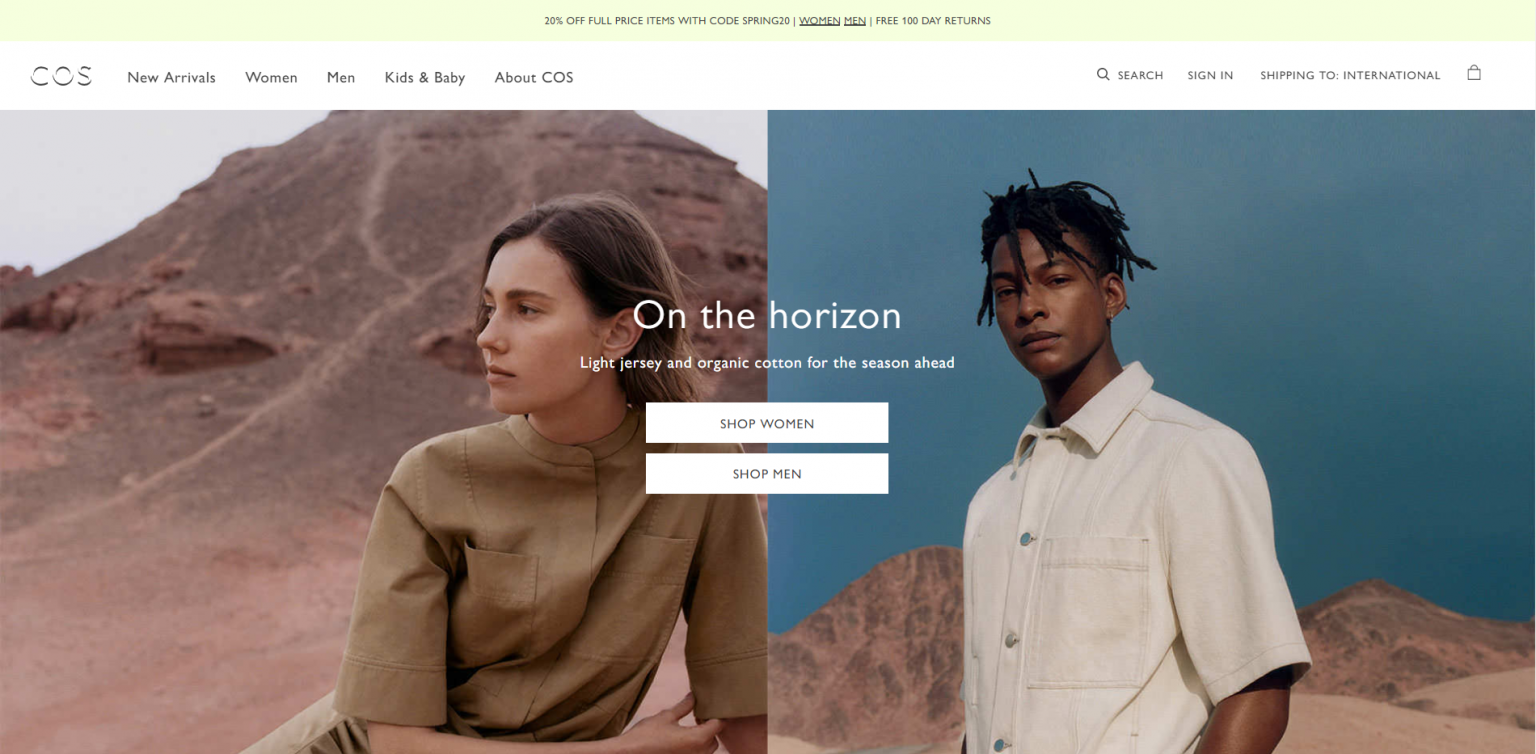This is a screenshot from the clothing website "Kos." The screenshot does not contain any menu bar or indication of the computer type, whether Mac or PC, on which it was taken.

The upper portion of the screenshot features a light neon yellow bar that announces a promotion: "30% 20% off full price items with code SPRING20." Additional information includes options for "Women," "Men," and "300-day returns."

Below this, there is a slightly wider white menu bar with the following items from left to right: 
- The logo of the store "Kos" in embossed white and black lettering
- Menu options: "New Arrivals," "Women," "Men," "Kids and Babies," "About Kos"
- A blank space
- A magnifying glass icon followed by "Search," "Sign In," "Shipping to International," and a shopping cart icon

Underneath the menu bar, the main content consists of two side-by-side photos. On the left, there is an image of a woman sitting in front of a hill made of redstone. She is wearing a khaki green top with quarter-length sleeves and two breast pockets. She has short brown hair and is looking over her right shoulder. The right photo features a man with slightly long black hair standing in front of the same redstone background. He is wearing a white button-up shirt with a collar and silver buttons.

Overlaying the two images, in white text, are the words: "On the horizon: light jersey and organic cotton for the season ahead." Below this text, there are two white rectangular buttons with blue lettering, labeled "Shop Women" and "Shop Men."